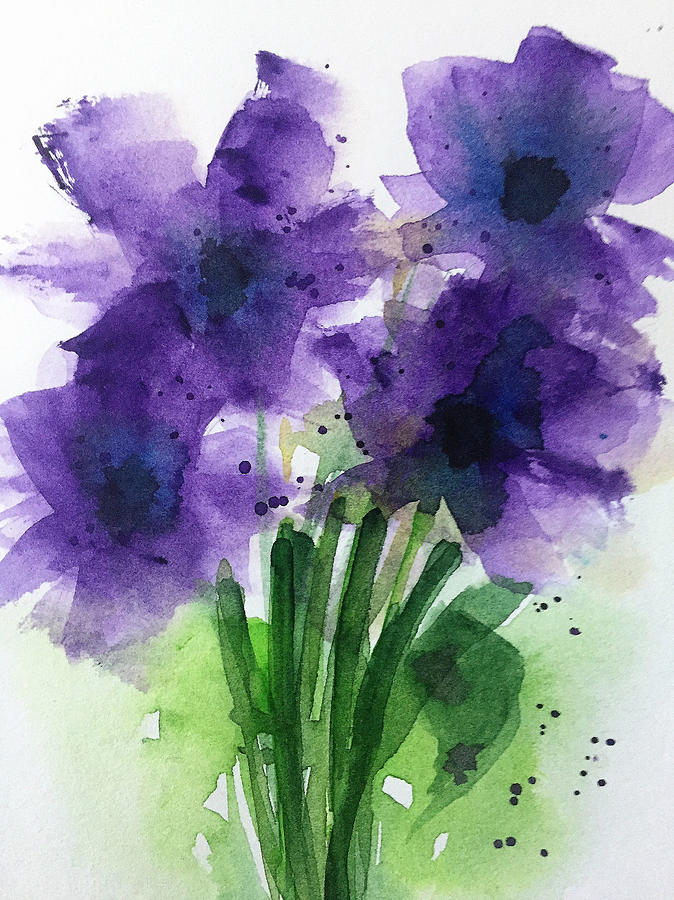This vertical, rectangular watercolor painting on white paper features a cluster of at least seven green stems rising from the center, each supporting four prominent dark purple flowers with black centers. Surrounding the flowers and stems is a subtle wash of faded green, giving an impression of foliage or grass. The purple flowers occupy both the top and central sections of the image. Tiny black dots are scattered throughout the painting, reminiscent of larger, rounder pepper flakes, particularly around the flowers and falling towards the lower right corner, where a slight bluish tint emerges from the otherwise white background. The painting exhibits a spongy, less defined style with lighter purples and greens blending around the main subjects, giving it a crude yet ethereal quality.